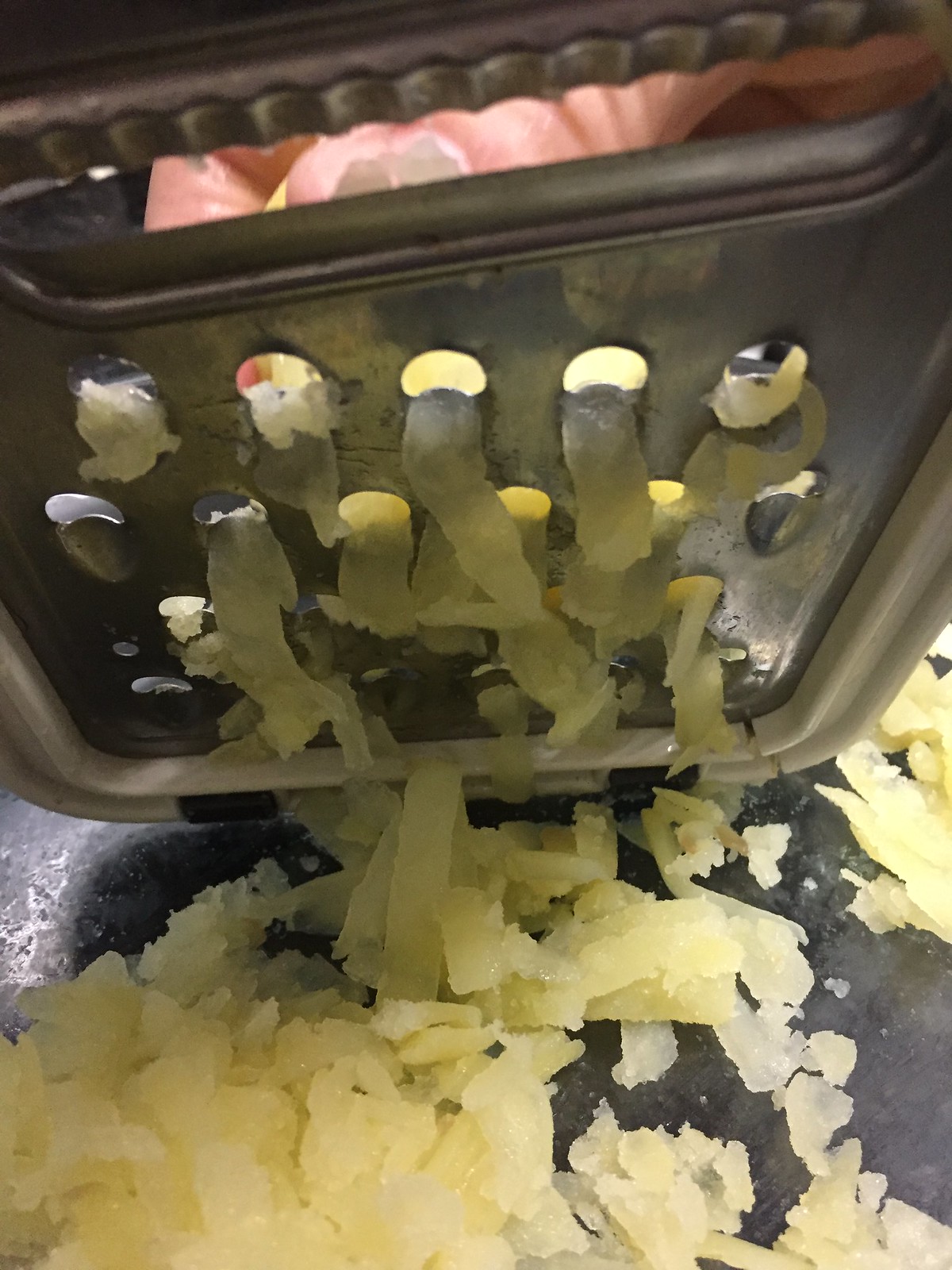This is a close-up photo capturing the intricate process of cheese being grated with a metallic box grater. The grater, which has a white plastic edge, appears aged and well-used. The person grating, likely Caucasian, is partially visible at the top, with just a bit of their hand and fingers in view. The cheese being shredded is a creamy, whitish-yellow color, possibly Parmesan or mozzarella, and is emerging from almost all the holes of the grater. The cheese's texture appears somewhat rough and gooey as it falls, forming a small, irregular pile on a flat, dark countertop beneath. Shadows cast on the grated cheese add depth to the image. The photo, taken either with a personal camera or a cell phone, provides an intimate and detailed look at this everyday kitchen activity.